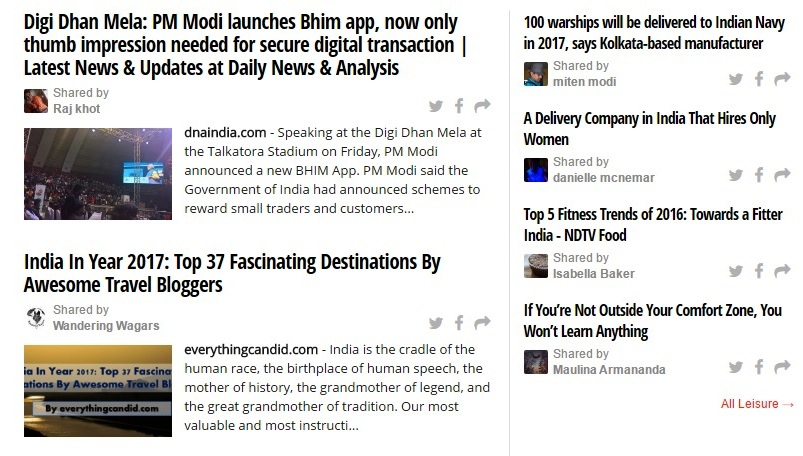This image features excerpts from news articles, likely displayed on a digital news platform where users can click to read the full content. On the left, there is an article titled "PM Modi Launches BIM App: Now Only Thumb Impression Needed for Secure Digital Transactions." The snippet explains that Prime Minister Modi made this announcement at the Digidhan Mela held at Tora Stadium on Friday, emphasizing the government's schemes to reward small traders and customers. This article is sourced from Daily News and Analysis, indicated by the tag DNAIndia.com.

Below this, another article is visible, focusing on travel. Titled "India Among 2017’s Top 37 Fascinating Destinations by Awesome Travel Bloggers," this piece is sourced from everythingcandid.com. It highlights India’s rich cultural heritage, describing it as "the cradle of the human race, the birthplace of human speech, the mother of history, the grandmother of legend, and the great grandmother of tradition." However, the last part of the excerpt is cut off.